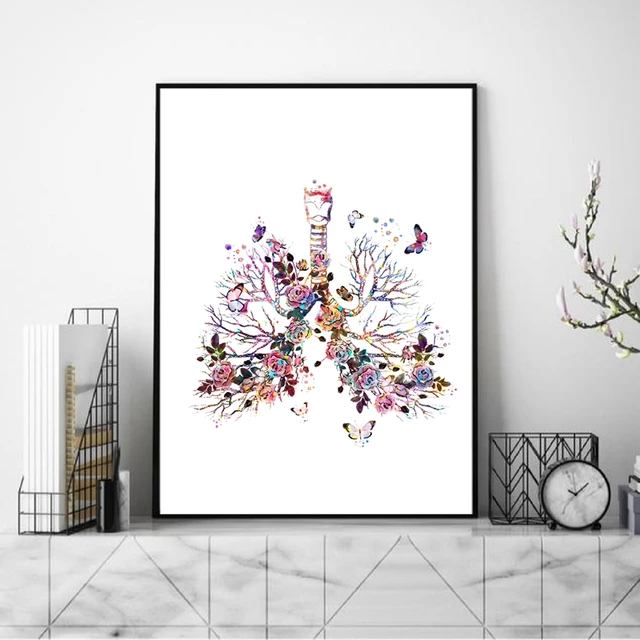In a modern office setting, a meticulously designed workspace centers around a striking piece of art. This art piece, framed in black with a white background, showcases a vibrant, multicolored depiction of a flowering bush adorned with butterflies, featuring hues of pink, purple, blue, green, and white. The artwork sits prominently on a sleek marble shelf against a dark gray wall.

Beneath this shelf, a white table with geometric grooves stands out. On the table, to the left, is a wire basket containing files and papers, positioned next to a smaller black cylinder and a white cylinder. To the right, another wire basket holds additional files, accompanied by a small black-and-white alarm clock and a stack of papers. An indoor plant branch extends into the scene, adding a natural touch.

Overall, this image encapsulates a harmonious blend of organizational elements and artistic flair, highlighted by the colorful and detailed centerpiece painting of a flowering bush and butterflies.